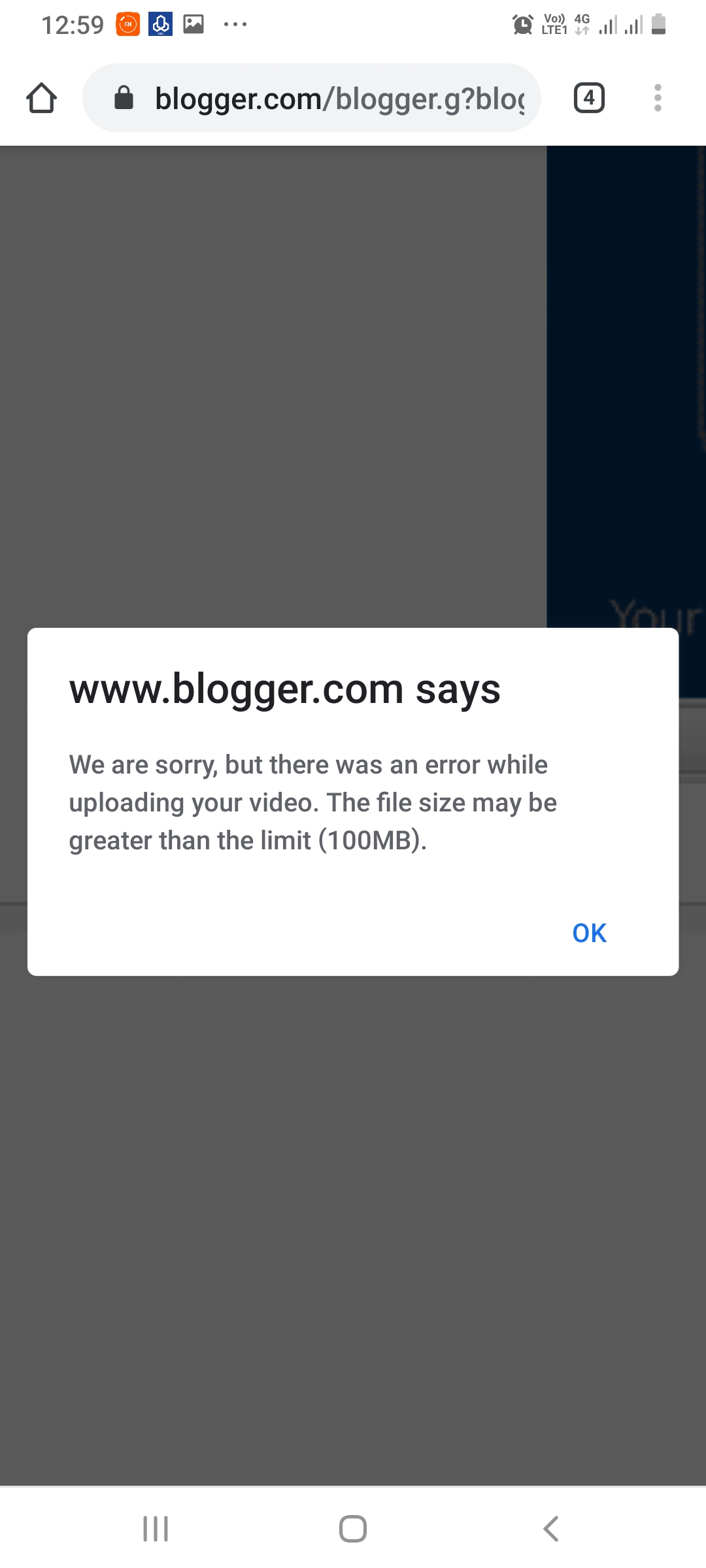The image depicts a smartphone screenshot captured at 12:59. It shows the screen while browsing the website blogger.com, specifically the URL "blogger.com/blogger.g?blog". The user has four tabs open, although only one tab is visible in the screenshot. The visible web page has a gray background with some elements highlighted in blue. Dominating the screen is a pop-up message from www.blogger.com stating: "We are sorry, but there was an error while uploading your video. The file size may be greater than the limit (100 megabytes)." There is an "OK" button at the bottom of the pop-up for the user to acknowledge the message.